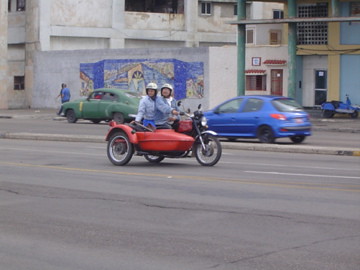In this slightly out-of-focus city street scene, a blocky, gray concrete building with scattered windows dominates the left side, adorned with a blue and yellow mural. In front of it, there are two parked cars—a vintage green vehicle from the 1950s facing the upper left, and a modern blue hatchback. On the right side of the picture, near a green building with tall pillars, a small motor scooter is parked. The focal point of the image is a three-wheel motorcycle with a red sidecar, carrying two individuals wearing jean jackets and white helmets, likely a man and a woman. They are driving towards the left, with the woman possibly seated slightly behind the man. The scene suggests a typical bustling road in Cuba, evidenced by the vintage cars and vibrant mural. Two people are also visible walking on the distant sidewalk, adding to the lively urban environment.